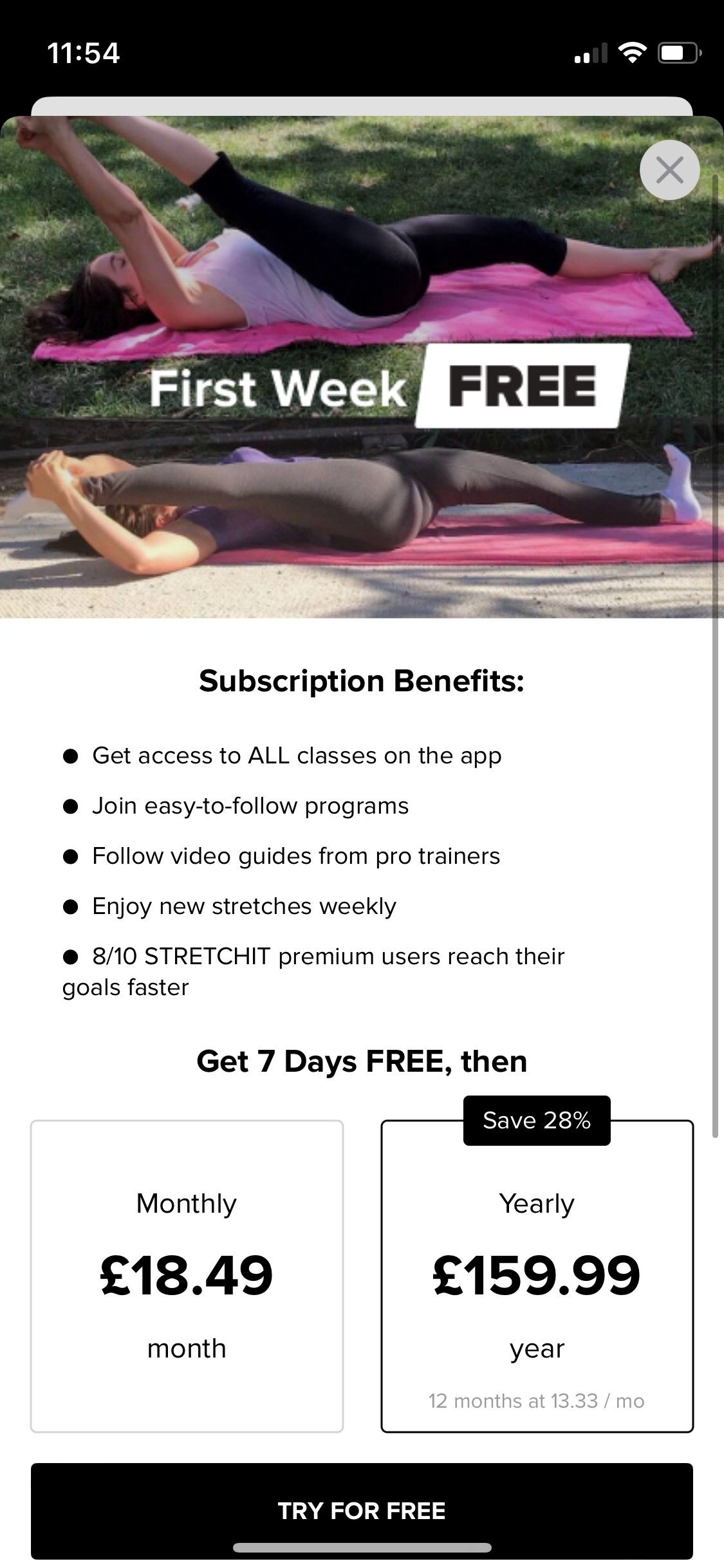The screenshot displays a promotional interface from an app on an iPhone. 

In the top-left corner, the device's time is shown as 11:54. The top-right corner includes the network signal bar, Wi-Fi icon, and a password field. The central portion of the screen showcases an advertisement with the caption: "First week free. Choose two ladies doing a yoga pose."

The promotional text highlights subscription benefits, stating: "Get access to all classes on the app. Join easy-to-follow programs. Follow video guides from pro trainers. Enjoy new stretches weekly." 

There's also a mention of statistics: "Over 10 Stretch-It Premium users reach their goals faster."

Towards the bottom of the screen, a pricing summary is provided: "Get seven days free. Then save 28% yearly, £159.99. Monthly, £18.49 per month."

At the very bottom of the screen, a button prompts the user with "Try it out for free," located above the navigation bar specific to iPhones.

The colors utilized in the interface include pink, black, white, green, and gray, all set against a predominantly white background.